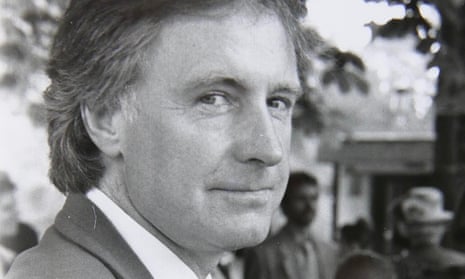This black-and-white photograph, rectangular with a width twice its height, prominently features a man visible from the shoulders up in the foreground. He is wearing a business coat and a collared button-up shirt, his short, dark-colored hair neatly in place. The man’s body is oriented towards the right while his face tilts slightly towards the bottom right corner, yet his eyes engage directly with the camera ahead. His expression is a mix of seriousness and a subtle smirk. Behind him, the image softly blurs into a backdrop of multiple out-of-focus figures, including a man in a suit and tie and another wearing a hat. Distant trees and a low, single-story building add depth to the scene, confirming the outdoor setting. The overall aesthetic and design of the photograph showcase a harmonious blend of the man’s poised presence against a busy yet indistinct background.